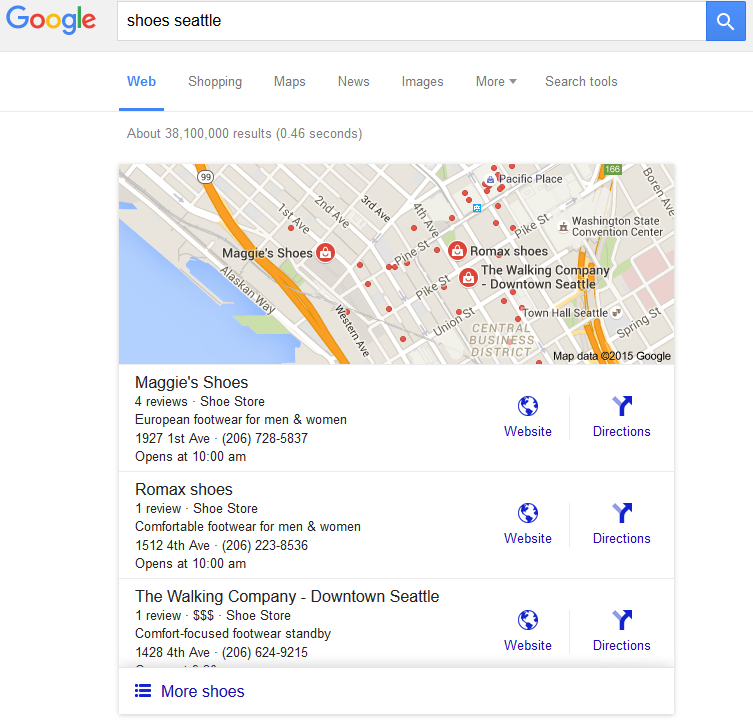A detailed screenshot of a Google search for "shoes in Seattle" displays the familiar Google homepage with its multicolored logo on the left side of the white search bar. The search results have populated with approximately 38,100,000 entries. At the top right of the search bar, there is a blue magnifying glass icon where the user initiated the search. The results include a small map showing shoe store locations in Seattle and a vertically listed snippet featuring three shoe stores: Maggie's Shoes, Romax Shoes, and The Walking Company in downtown Seattle. At the bottom of the screenshot, there is a white bar labeled "More shoes," suggesting additional stores can be viewed by clicking on it. The intent of the search appears to be for someone needing to buy shoes and exploring their options through Google.